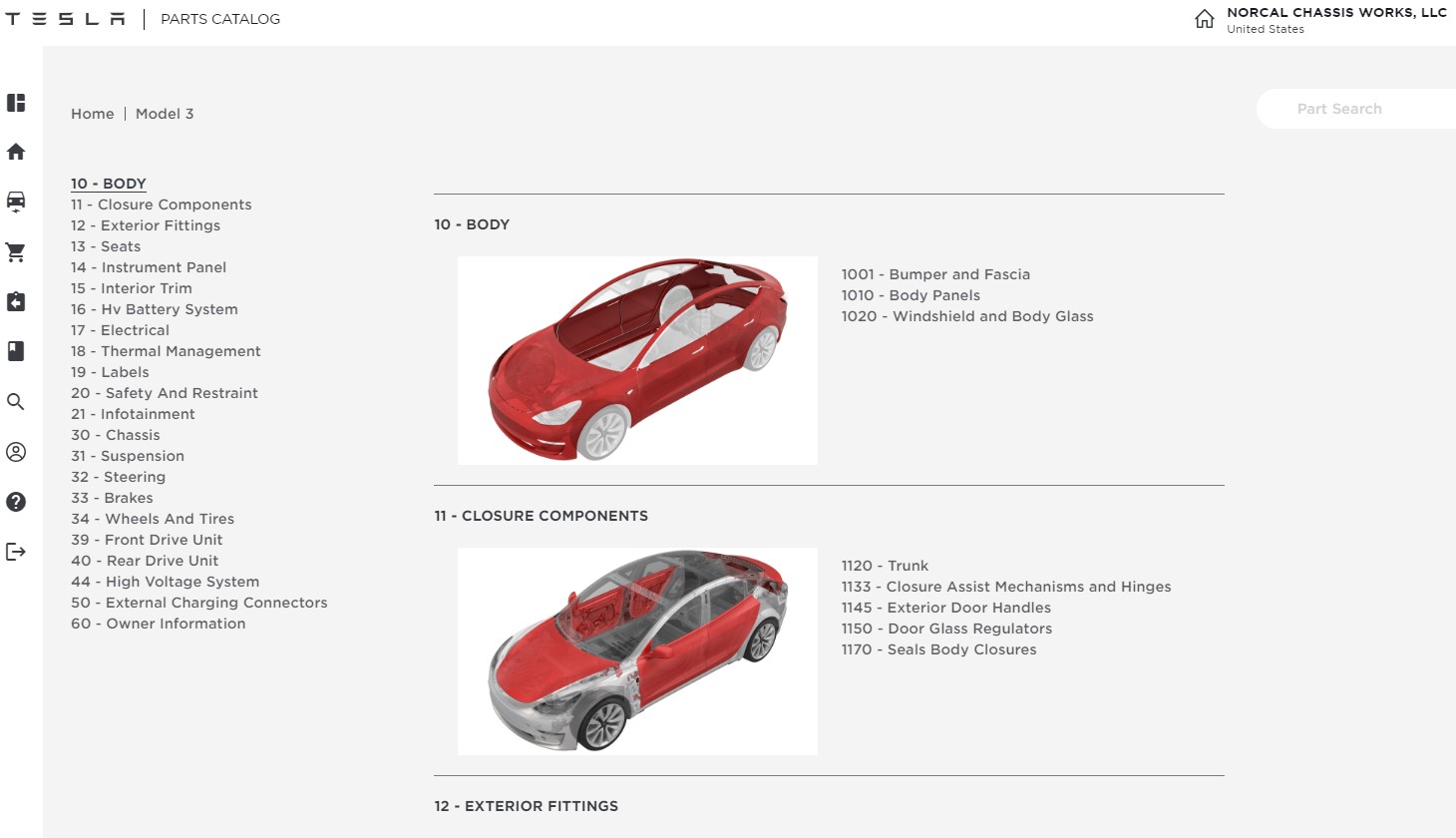This image depicts a screenshot of the Tesla Parts Catalog website, specifically focusing on the body parts for the Tesla Model 3. The central part of the screen features two detailed illustrations of car components. 

The first illustration, predominantly in red, showcases an incomplete Tesla Model 3, highlighting various parts such as the open roof, a single visible seat, bumpers, fascia, body panels, windshields, and body glass. It provides an intricate view into the structural elements still under assembly.

The second illustration focuses on closure components, displaying parts like the trunk, closure assist mechanisms, hinges, exterior door handles, door glass regulators, and seals for body closures. These parts are essential for the exterior fit and finish of the vehicle.

Below these sections, another illustration displays, this time in red and silver, labeled as "Exterior Fittings," although the website cuts off, making further details of this section unclear.

In the upper right corner of the screenshot, the site is identified as NorCal Chassis Works, LLC, United States, and includes a small home icon, a part search function, and "Tesla Parts Catalog" as navigational elements. The left side of the website lists various body parts, numbered 11 through 60, while vertically aligned images present additional visual information about the parts catalog.

Overall, this screenshot effectively captures a detailed and organized layout of Tesla Model 3 body parts available for search and review on the Tesla Parts Catalog website.